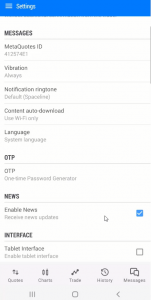In this detailed image, we observe a smartphone screen with various settings and options displayed. At the top of the screen, highlighted in blue, is the "Settings" section. Below it are various settings such as "Messages" with a sub-option for "Message Codes" set to 10. The "Vibration" setting is enabled to "Always," and the "Notification Ringtone" is set to the default sound. 

The settings continue with "Font" set to "Space" and "Content Auto Download" restricted to usage over Wi-Fi only. Below these, the "Languages" setting indicates the "System Language" is configured. The "One Time Password (OTP) Generator" option is visible as well.

Further down, there's a setting for "News" where "Enable News" is checked to receive news updates. Under the "Interface" category, the "Tablet Interface" option is available but not enabled.

Towards the bottom, there are tabs labeled "Quotes," "Charts," "Trade," "History," and "Messages," indicating different sections of an app. At the very bottom of the screen, we see the navigation keys typical of an Android mobile device: the recent apps key on the left, the home key in the middle, and the back navigation key on the right.